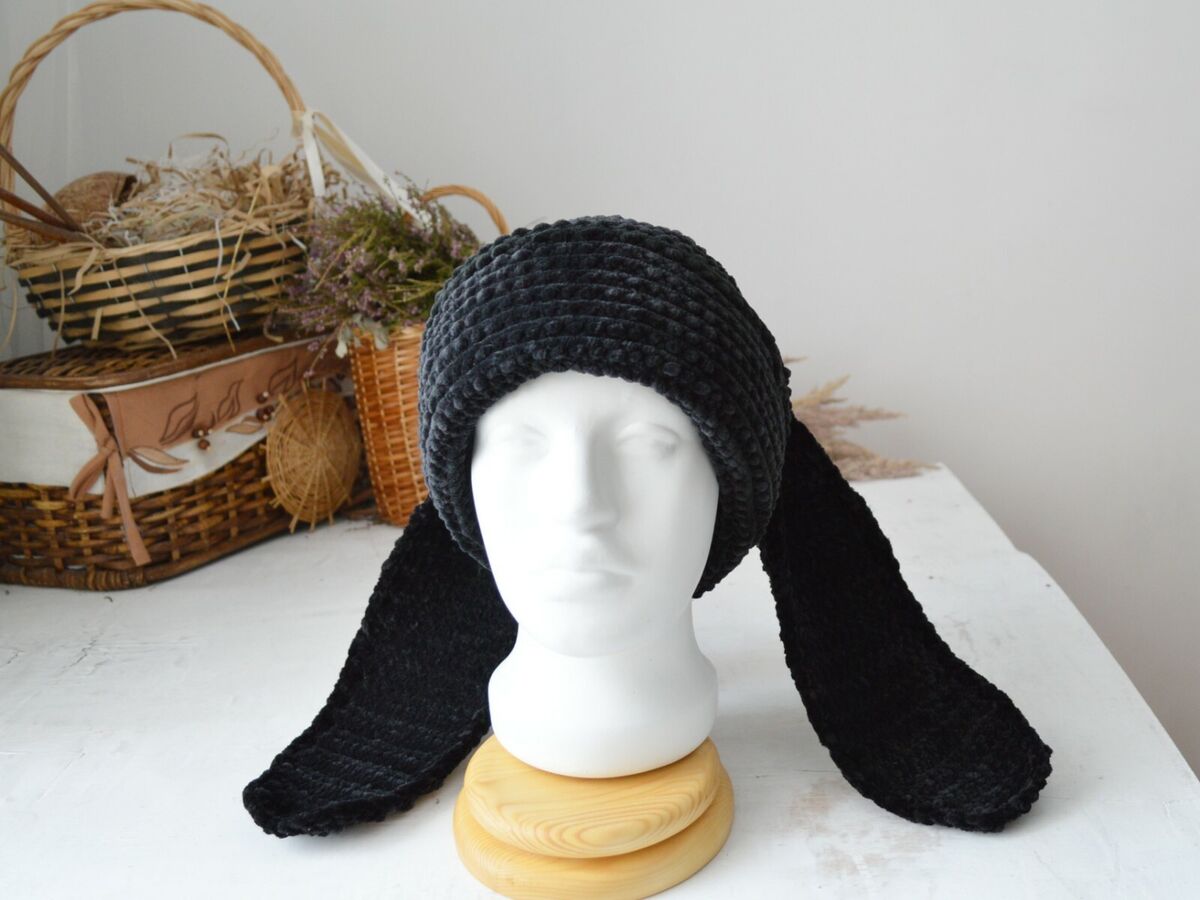In the image, a white mannequin head is adorned with a dark blue, hand-knit toboggan featuring long, hanging pieces that resemble bunny ears. The toboggan and its extended parts appear to be crocheted from yarn, giving it a textured look. The mannequin is mounted on a tan head holder atop a white table. The setting seems to be someone’s home, indicated by the background elements—a few wicker baskets filled with straw and greenery that serve as decorations. These are placed against a grayish-tan wall, adding earthy tones to the composition. The mannequin’s facial features like eyes, nose, and lips are clearly visible, adding to the detailed presentation of the toboggan. The absence of text in the photo emphasizes its focus on showcasing the handcrafted product in a cozy, rustic environment.